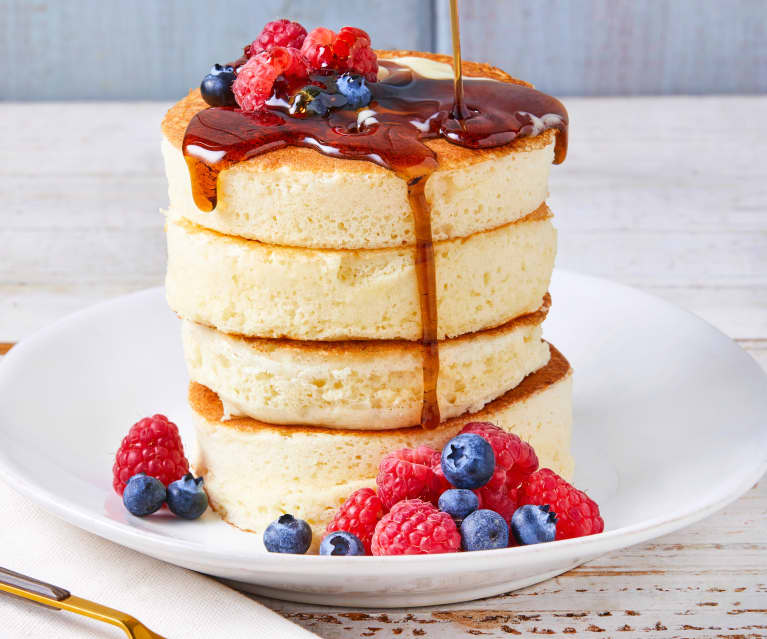In this photograph, four thick and small pancakes, each about two inches tall, are stacked neatly on a white plate with slightly raised edges resembling a flat bowl. The plate is placed on a whitewashed wooden table with a blue-grayish wooden background. Surrounding and atop the pancakes are a scattering of fresh raspberries and blueberries, with golden syrup being poured over the top pancake, creating a tantalizing drizzle down the sides. A pat of butter melts atop the stack, blending into the syrup and berries. Partially visible in the foreground is the handle of a gold utensil, either a fork or a spoon. The primary focus of the image is the delectable pancake stack accompanied by vibrant berries and gleaming syrup.